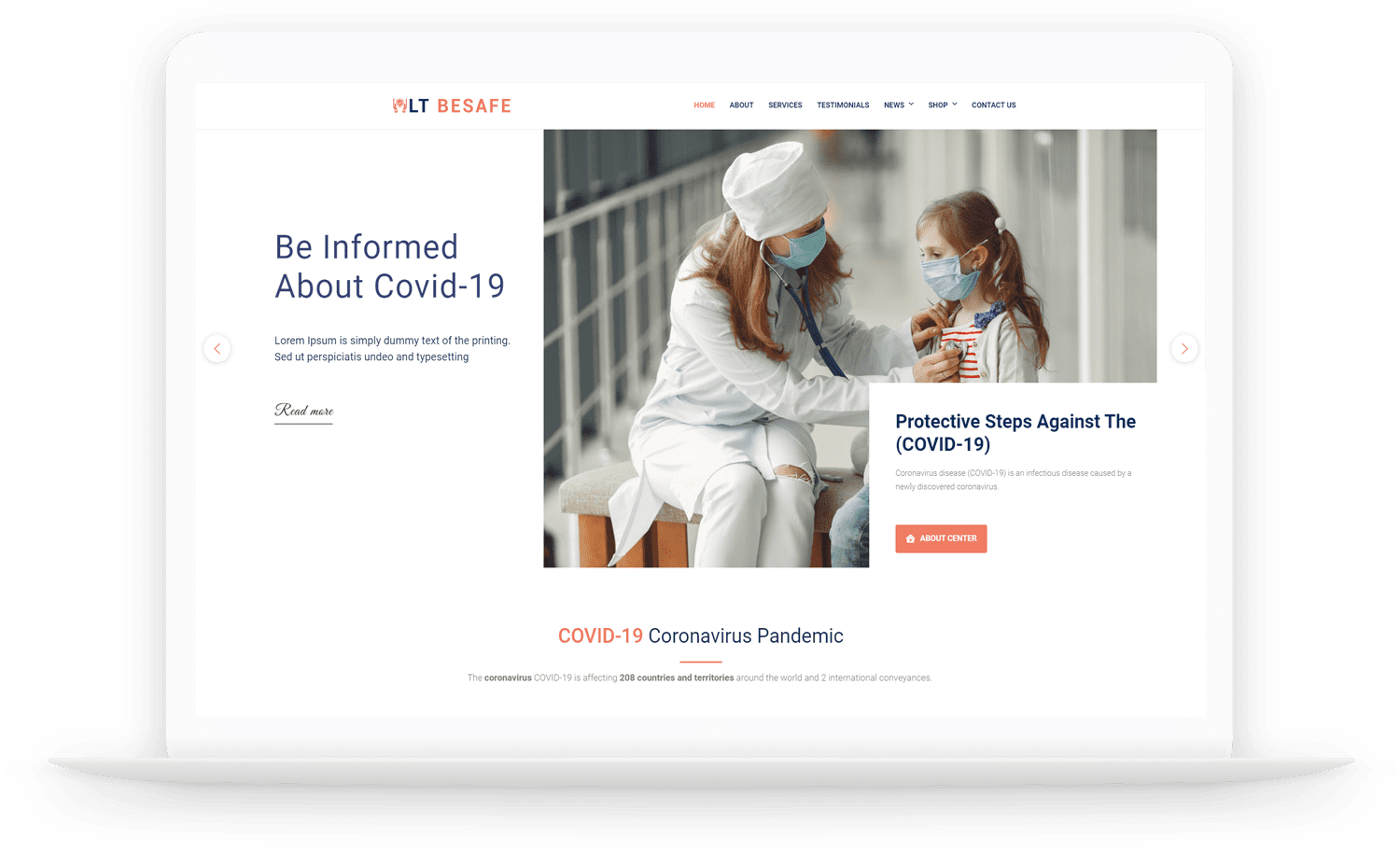In the image, we see a website interface titled "LCB Safe" displayed at the top left corner. The website features navigation links including Home, About, Services, Testimonials, Shop, and Contact Us. Central in the image is a scene where a nurse, dressed in a white uniform and wearing a nose mask, is attending to a young girl who is also in white and wearing a nose mask. The nurse appears to be listening to or monitoring the girl's heartbeat with a stethoscope. 

Embedded within the image is informational text about COVID-19, detailing its impact and preventive measures. It highlights that COVID-19 is an infectious disease caused by a newly discovered coronavirus and emphasizes protective steps against the virus. There is a note mentioning that the coronavirus pandemic has affected 208 countries and territories, as well as international conveyances.